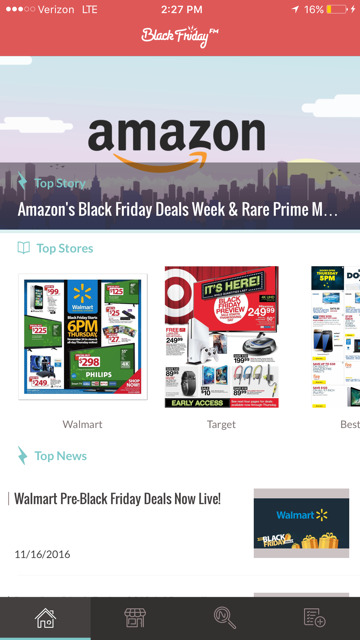The image depicts a screenshot from the Amazon app during the Black Friday event. At the top of the interface, there is a prominent header with a peachy red background. Centered within this header, decorative cursive text in white reads "Black Friday", accompanied by three dynamic sparks emitting from the word "Friday", reminiscent of fireworks or candles. A trademark symbol is positioned at the top right of this text.

Below the header, the background transitions into a cloudy sky, with the iconic Amazon logo prominently displayed. The logo features the text "amazon" in a traditional black font, with the characteristic upward-curved arrow beneath the letters.

The bottom portion of the image showcases a cityscape. Overlaid on this is a dark gray background featuring various elements. In the top left corner, a teal lightning bolt icon labeled "Top Story" catches the eye, followed by the white text "Amazon's Black Friday Deals Week" in a bold and capitalized format, with an ellipsis trailing a capital "M."

A thin blue line acts as a divider below this text. On the left bottom, there's a blue icon of an open book, indicating "Top Stores." Next to this, left-aligned, there's a sequence of promotional flyers: the first for Walmart, labeled in small gray text, followed by a flyer for Target with similar small gray text identification. To the far right, only half of a flyer is visible, but the fragment of the word "Best" in gray clearly identifies it as a Best Buy advertisement.